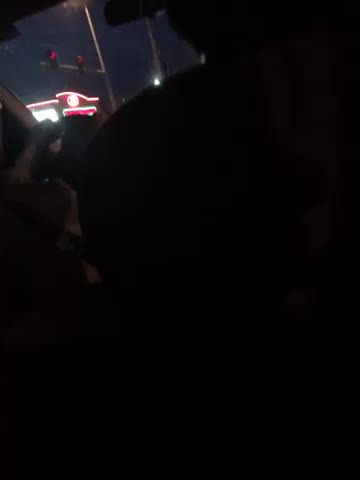This image is taken from the backseat of a car at night, and it is extremely dark. The background is almost entirely black, making it difficult to discern details at first glance. However, in the upper left-hand corner, there is a faint image featuring small red and white lights. These could be part of a red sign from a building or restaurant off to the side of the street, contributing a feeble glow against the dark setting. 

In the dim light, you can vaguely see two hands gripping a steering wheel, hinting that there is a driver, although their features are not clearly visible. The photo also captures the back of the passenger seat, though it's unclear if anyone is seated there. Through the windshield, there's a lit-up restaurant or building, adorned with red lights and a red sign. Additionally, traffic lights can be glimpsed, casting a red hue perpendicular to the car, alongside various street lights. This all underscores the nocturnal ambiance, further highlighted by a glowing light near the restaurant, persistently outlining the night sky.